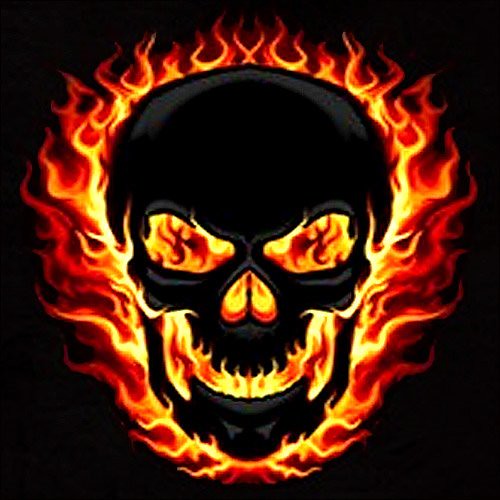This striking image features a black skull set against a deep black background. The skull is intricately outlined and filled with dynamic flames, creating a dramatic visual effect. The fiery outline is particularly prominent on the sides, tapering at the top and bottom. The flames transition from yellow to deep orange and red, becoming darker towards the outer edges. In the eye sockets, the flames form sideways, rounded triangles that darken from a deep red at the center to brighter yellows and oranges. The nose of the skull, shaped like an upside-down heart, is also filled with flames, as is the mouth, which gives the appearance of a fiery smile. The vivid flames contrast sharply with the dark skull, making the entire image both haunting and mesmerizing.